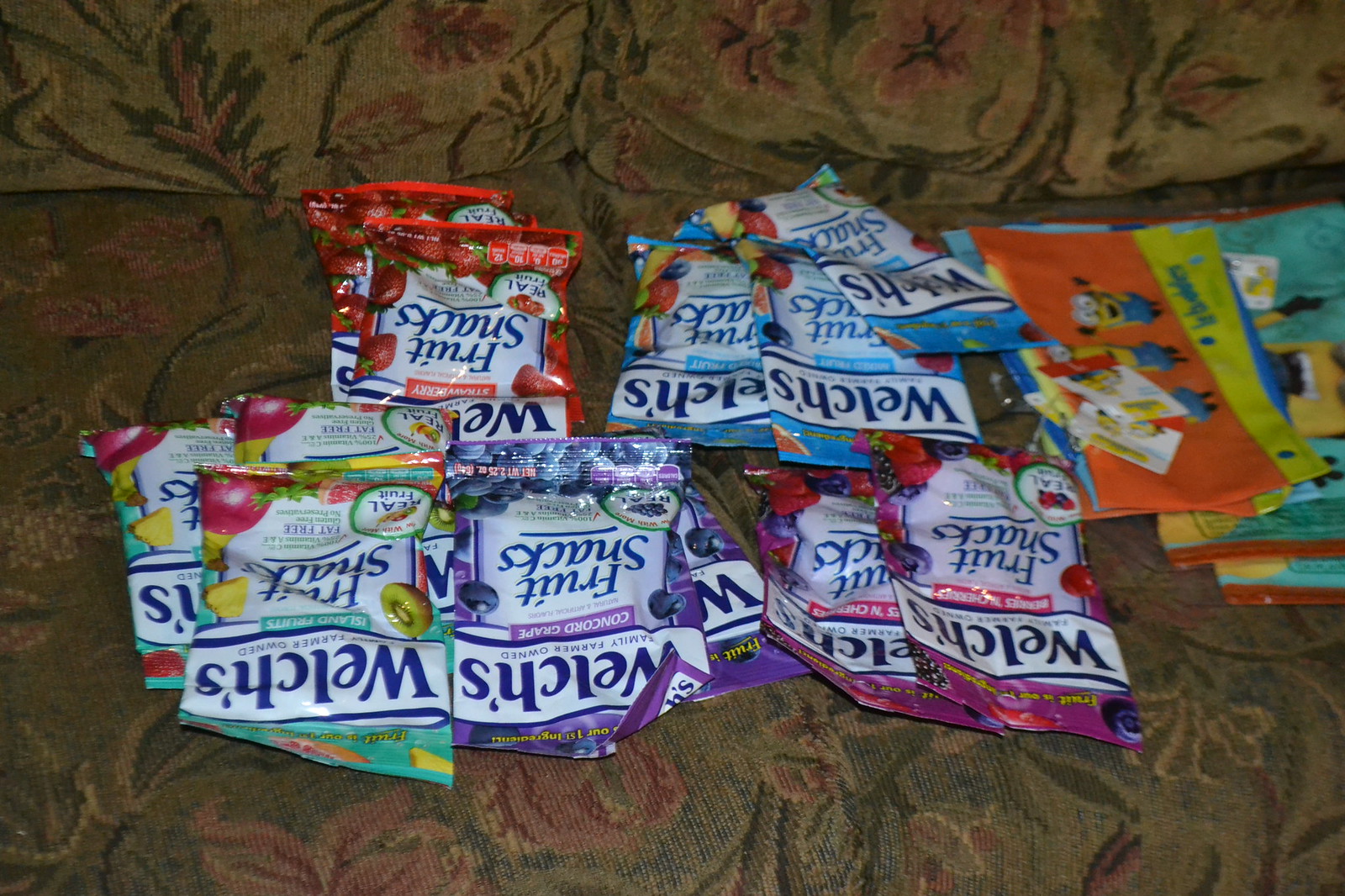This detailed photograph showcases an assortment of Welch's fruit snacks arranged on a brown sofa adorned with a floral motif, featuring light pink and yellow flowers with green leaves. The fruit snacks are meticulously separated into five distinct piles, each containing two to three packets. The packets are grouped closely together, almost overlapping, and are positioned upside down from our viewpoint, making them a bit challenging to read.

In the front row, to the left, the Island Fruits packets display a mix of fruits like kiwi, pineapple, and possibly grapefruit. The center pile features the Concord Grape flavor, easily identified by its purple packaging decorated with grapes. To the right, the Berries and Cherries packets highlight a variety of berries, including blueberry, cherry, strawberry, and possibly blackberry. In the back row, the Mixed Fruit packets, with a blue packaging, seem to depict peach, blueberry, strawberry, and maybe mango or raspberry. On the top left, the bright red Strawberry packets are covered with strawberry images.

Adjacent to these fruit snack piles, a collection of pouches or bags flaunt colorful designs predominantly featuring yellow cartoon characters in overalls, resembling Minions. The entire setup suggests a lively preparation, possibly for a gathering or a children's event.